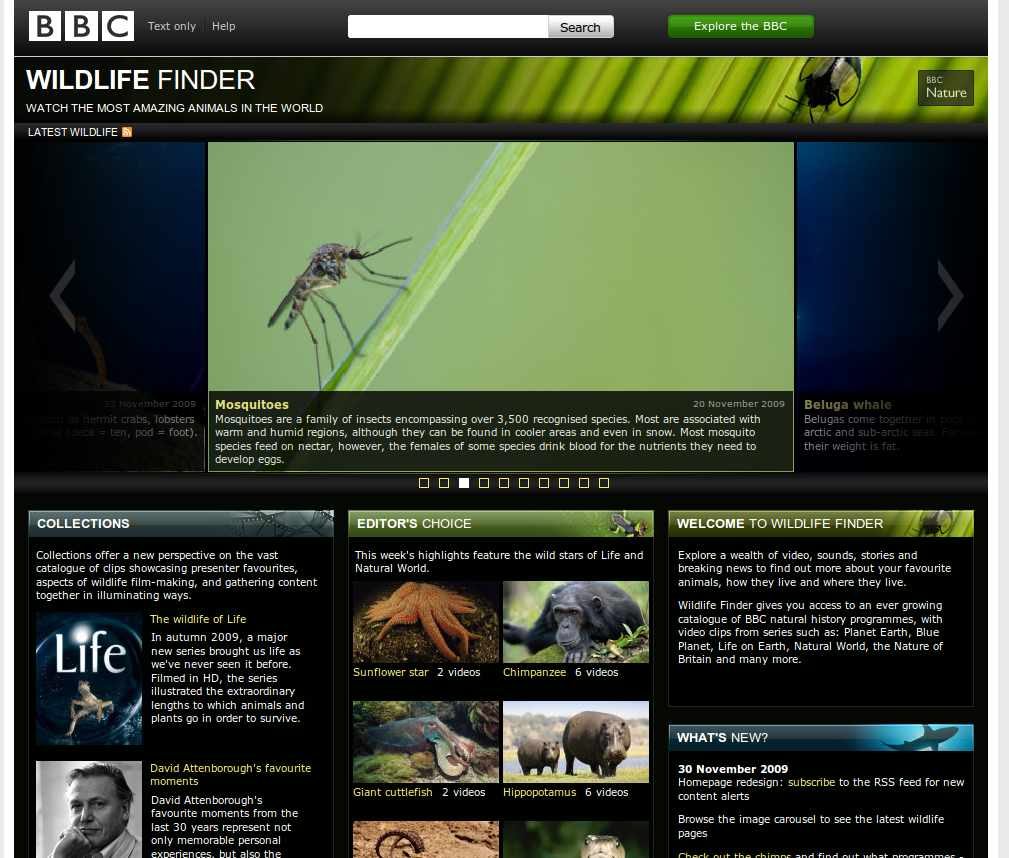This is a detailed caption for an image from the BBC Wildlife Finder page:

---

The screenshot is from a BBC website page dedicated to wildlife. At the top, a black ribbon spans the width of the screen. Situated in the upper left corner is the iconic BBC logo, displayed in white boxes with bold black capital letters. To the right of the logo, small white text reads "Text Only," followed by "Help." Next to these options is a white search bar, and further to the right, a dark green button with white text invites users to "Explore the BBC."

Below this header, the phrase "WILDLIFE FINDER" appears in bold white capital letters, with "Wildlife" further emphasized in a heavier font weight. Beneath this, in smaller white text, it reads, "Watch the most amazing animals in the world." Following this, the term "LATEST WILDLIFE" appears in the same small white text.

Centered on the page is an image of a mosquito perched on a green stem, set against a green background. Below this image, the word "MOSQUITOES" is presented in bold gold text. Underneath, smaller white text provides a detailed description: "Mosquitoes are a family of insects encompassing over 3,500 recognized species. Most are associated with warm and humid regions, although they can be found in cooler areas and even in snow. Most mosquito species feed on nectar; however, the females of some species drink blood for the nutrients they need to develop eggs."

This mosquito image is placed within a smaller box, flanked on either side by a navy bluish-black background featuring forward and backward arrows for navigation.

Below this box, the content is divided into three columns, each introduced by a ribbon indicating its category. The first column is labeled "Collections" with a light gray ribbon. The second column, marked "Editor's Choice," has a green ribbon. The third column, titled "Welcome to Wildlife Finder," also features a green ribbon. Each column contains content relevant to its category.

---